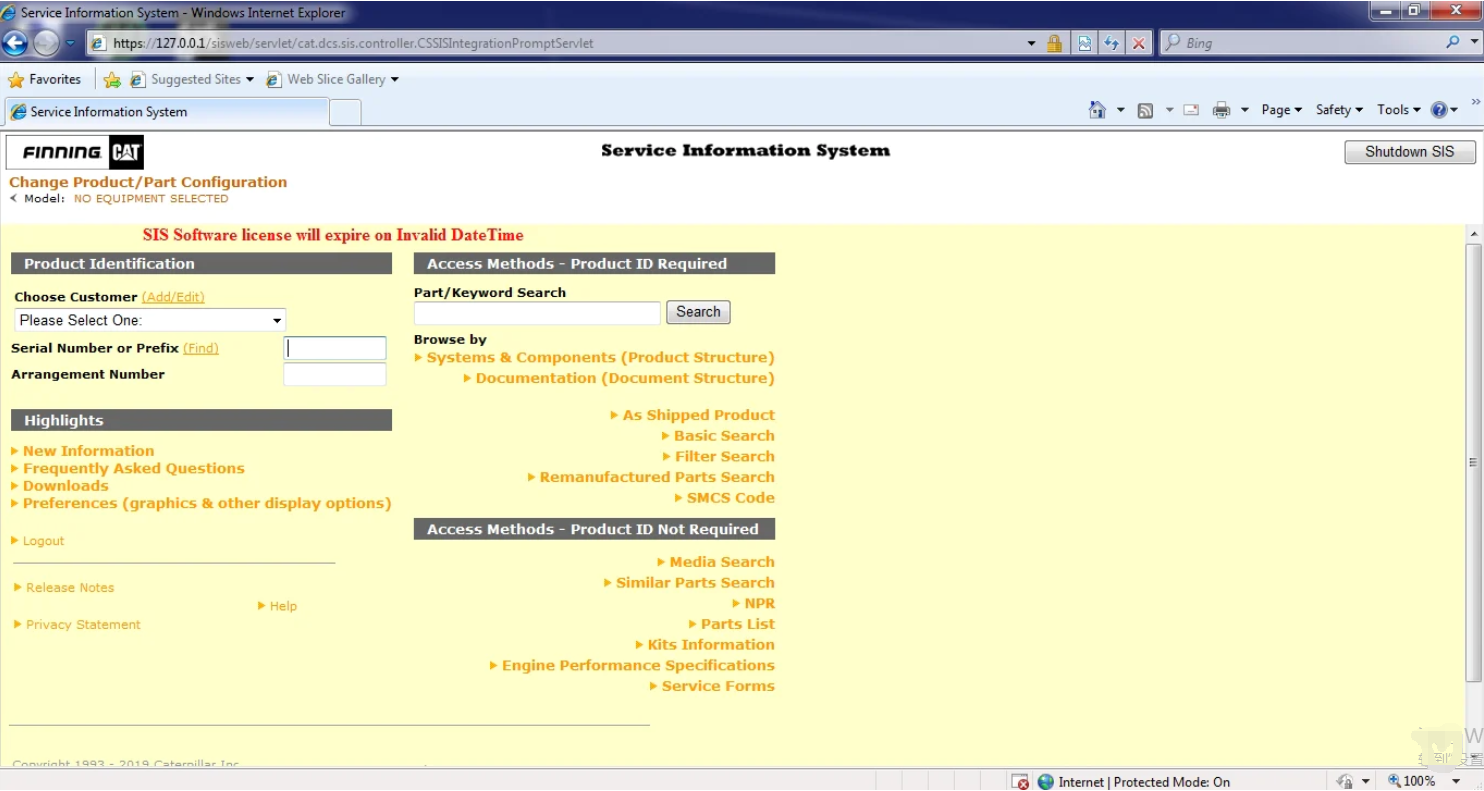The image depicts a website interface with extremely small print, making it difficult to read clearly. The page appears to be a "Service Information System" displayed in the Internet Explorer browser. In the search bar at the top, the term "service information system" is entered.

The website is associated with "FINNINA CAT," as noted prominently. Below the main header, there is an option to change the product part configuration, including a model number. The term "Service Information System" is repeated in a central location on the page.

On the right side, several icons are visible, alongside the text "shut down SIS in a box." Below this, highlighted in red text, is a warning that says, "SIS software license will expire on invalid date time." This warning is positioned on top of a golden box.

Additionally, the page features different sections delineated by gray bars. Some of these sections include "Product Identification," "Access Methods," and "Highlights." A detailed description is provided in gold lettering beneath each section. There are also fillable boxes available for user input related to product identification and access methods, with the note that product ID is not required.

Overall, the webpage is highly detailed, incorporating multiple interactive elements and important notices in various highlighted sections.